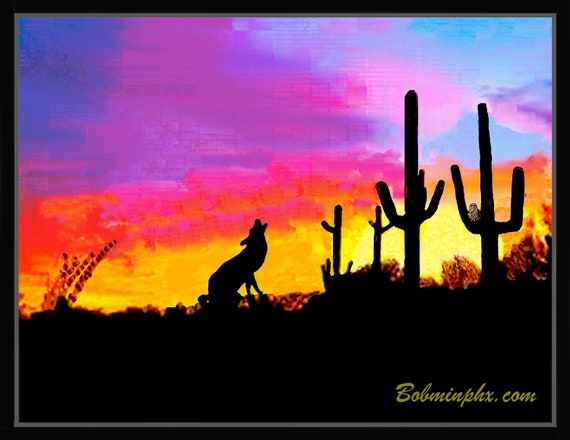This unique image resembles a postcard and depicts a dramatic desert scene at sunset. In the foreground, the silhouettes of four cacti and a howling coyote, or possibly a wolf, stand against the vibrant sky. The cacti and wolf are rendered entirely in black, adding to the striking contrast. The sky is an exquisite blend of purples, blues, pinks, reds, and yellows, with a small patch of blue at the top. The setting sun casts a mesmerizing array of colors across the horizon. The landscape also includes the outlines of tumbleweeds, additional desert plants, and trees in the background. Notably, an owl perches on one of the cacti. The image is bordered by a gray frame, and at the bottom, the website "bobmanphx.com" is prominently displayed in clean yellow text with a black outline, possibly indicating the artist or creator.